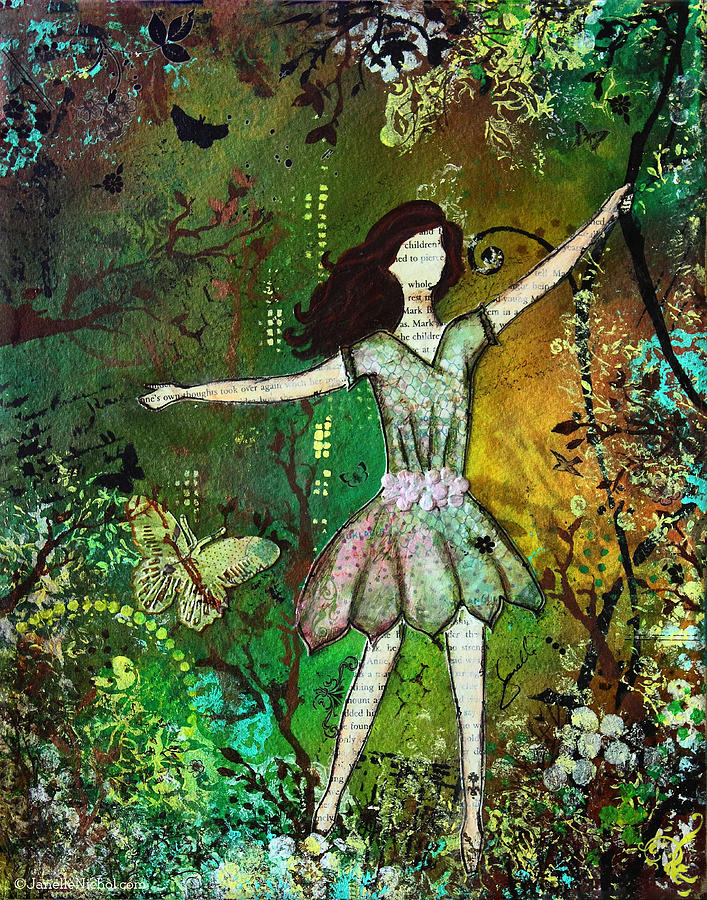This captivating and somewhat abstract painted image depicts a young woman standing in a dense, vibrant jungle forest. She has long, wavy dark brown hair and is grasping a black vine with her left hand, while her right arm hangs outward to her side. Her attire consists of a green dress adorned with a floral pattern, including a belt made of pink flowers. Remarkably, her skin is composed entirely of book text, giving her a unique texture with printed words that are visible but not legible, and she has no facial features or expressions. The background is a rich tapestry of lush foliage, various types of plant life, and vibrant colors including blues and yellows. Butterflies are scattered throughout the scene, with one large butterfly positioned near her floral skirt. The entire composition offers a mix of natural elements and artistic abstraction, blending the surreal nature of her text-laden skin with the dynamic flow of the jungle environment.